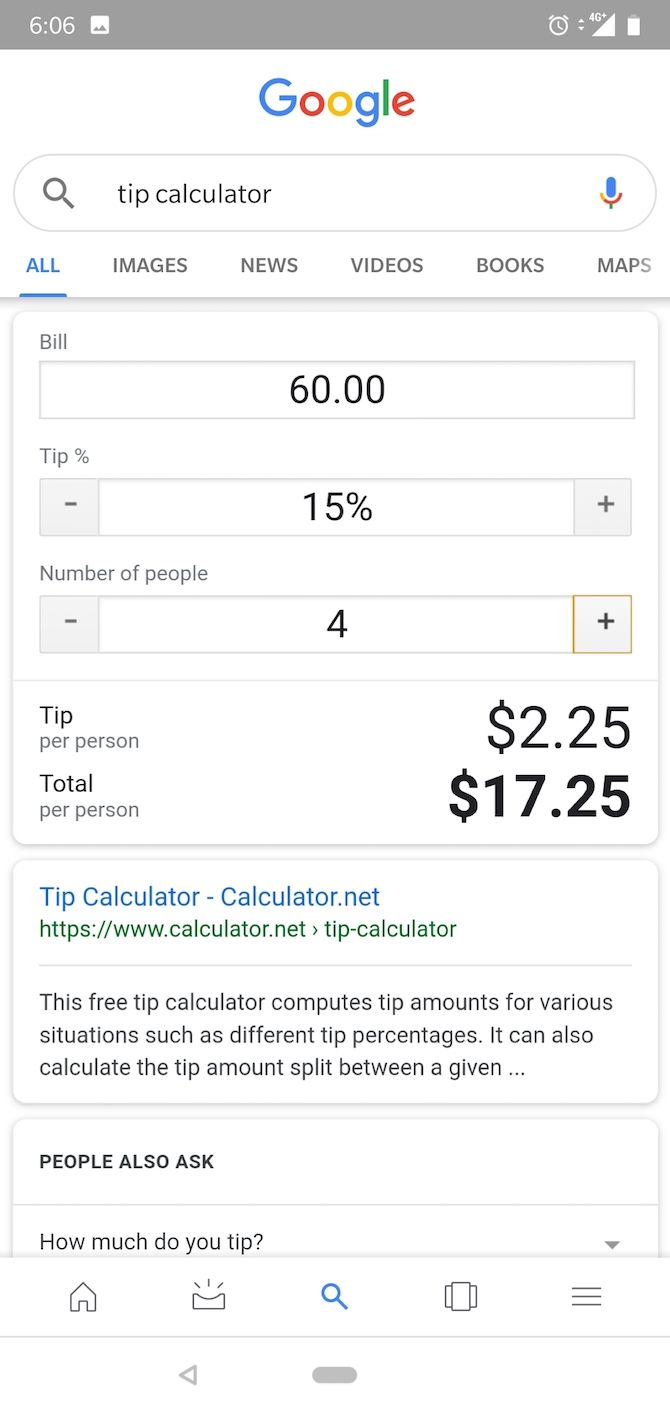Screenshot of a Google search result for "tip calculator." The page displays the usual Google navigation tabs, including "All," "Images," "News," "Videos," "Books," and "Maps." Below the search bar, there is an interactive result from TipCalculator.net. The tool allows users to input various details for calculating tips: 

1. The bill amount, which is set at $60.
2. The tip percentage, adjustable, currently set at 15%.
3. The number of people sharing the bill, which results in a tip per person of $2.25 and a total per person of $17.25.

The description notes that TipCalculator.net is a free tool designed to compute tip amounts for various scenarios and offers the ability to split the tip among a specified number of people. At the bottom of the page, there is a section titled "People also ask," featuring related questions, such as "How much do you tip?" The interface is user-friendly, providing a clear and handy resource for quickly calculating tips.